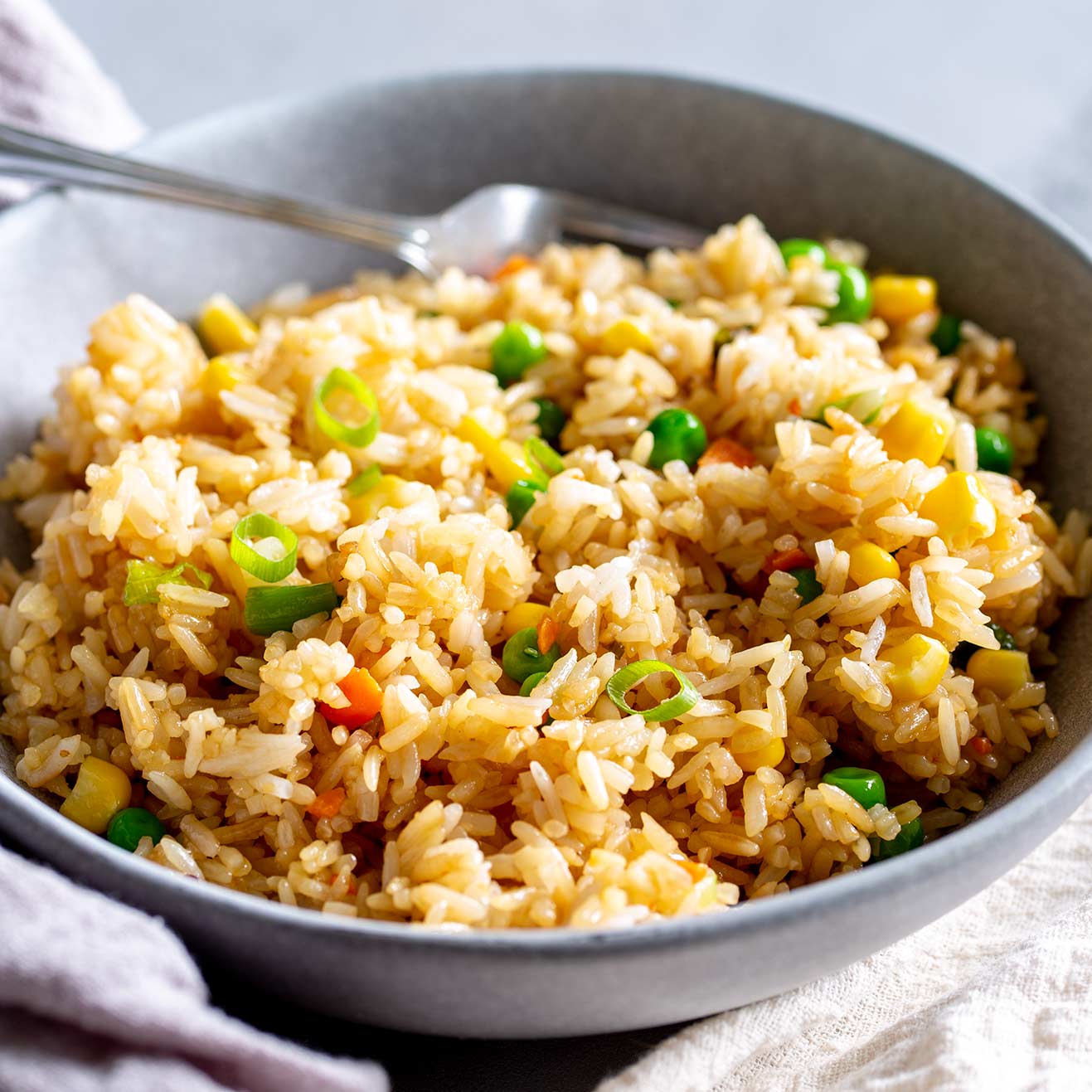A close-up image showcases a gray ceramic bowl positioned on a white tablecloth, filled with what appears to be a vibrant serving of fried rice. The bowl is placed towards the forefront of the image, emphasizing its textures and colors, while a silver fork is casually resting along the edge at the back. The foreground is sharply focused, highlighting the golden grains of rice, intermingled with an assortment of finely chopped vegetables. Bright orange carrots, tender peas, sweet corn kernels, crisp bell peppers, and delicate slices of green onions blend harmoniously throughout the dish, presenting a balanced mix of ingredients. The overall composition suggests that this appetizing fried rice, with its array of colorful veggies, is likely someone's savory meal, ready to be enjoyed.